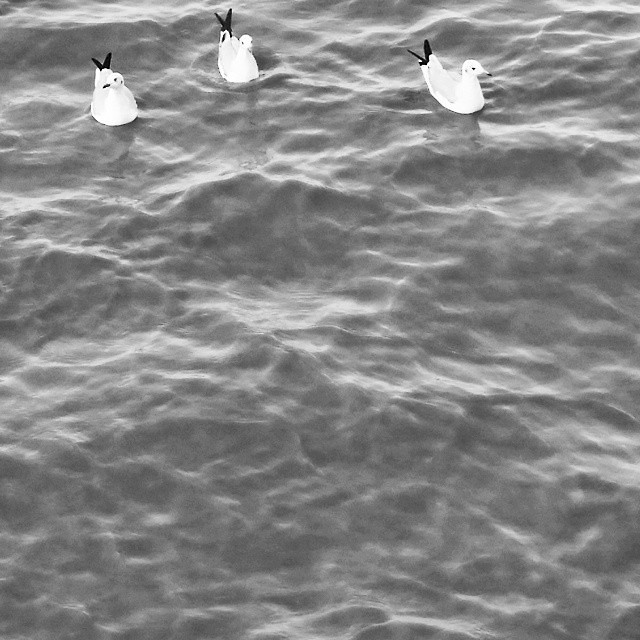This black-and-white photograph, though of poor quality and heavily grainy, evokes a poignant scene of three white birds, possibly ducks or seagulls, floating on wavy water. Captured from a high 45-degree angle, the birds swim towards the camera from the background, their positions dispersed from left to right across the upper portion of the frame. The image is notably overexposed, causing the birds' white bodies to blend into the bright water, while their dark tail feathers and beak tips stand in stark contrast. The water beneath them is marked by tire-like ripples and undulating waves, with reflections hinting at the presence of sunlight overhead. Despite the image's lack of color and clarity, the tranquil movement and positioning of the birds—each gazing in different directions—add a dynamic sense of life to the serene aquatic landscape.